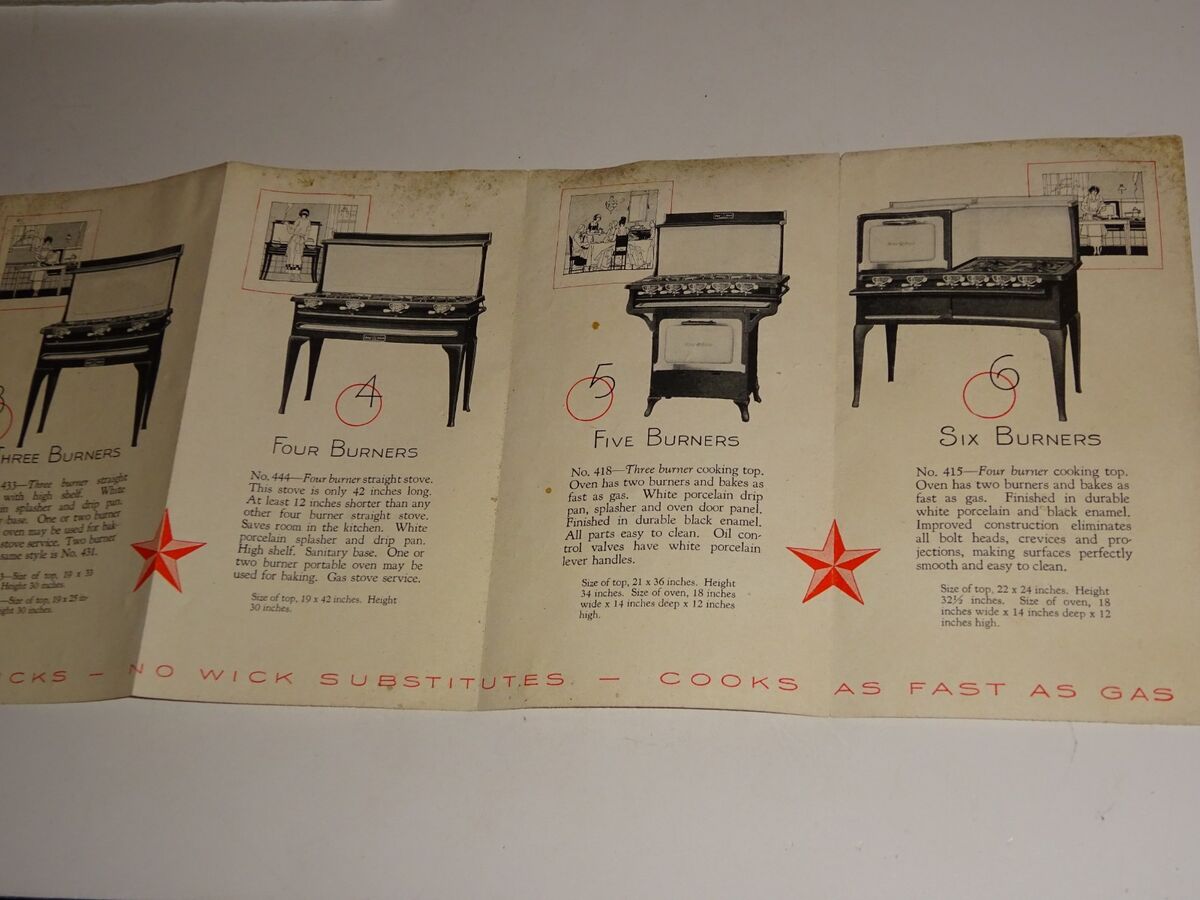This image features a weathered, yellowed catalog against a gray backdrop, showcasing a variety of vintage burner stoves from what appears to be the early to mid-1900s. The pamphlet is unfolded, displaying multiple panels that present stove models ranging from three to six burners. The stoves are depicted in both white porcelain and black enamel finishes, highlighting their improved construction designed for durability and easy cleaning. Each model is accompanied by descriptive text, listing features and emphasizing the efficiency of the stoves, stating "no wick substitutes cooks as fast as gas." A notable detail includes a red star separating the various sections of the pamphlet. The overall appearance of the catalog, with its browned and faded edges, suggests it has aged considerably over time, underscoring its historical significance.